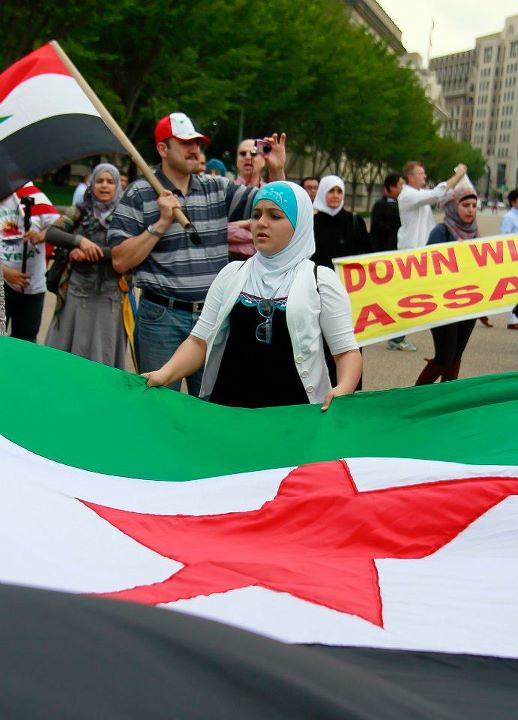The image captures a peaceful protest in the city streets, featuring approximately 15 demonstrators. Central to the scene is a man wearing a red and white baseball cap, sporting a dark and light gray striped collared shirt. He is holding a black, white, and red flag with a green star in the center, indicative of the Syrian flag. Another focal point is a woman holding one side of a larger Syrian flag; she is adorned in a headdress that is partly white and partly turquoise, a long-sleeved white sweater, a white vest, and a black dress, suggesting she might be Muslim. The protest appears centered around a banner with partially obscured text reading "Down With," speculated to target "Assassins." Surrounding the protestors are tall, green trees and buildings. Several people in the crowd are seen taking photos, amplifying the sense of a peaceful assembly.